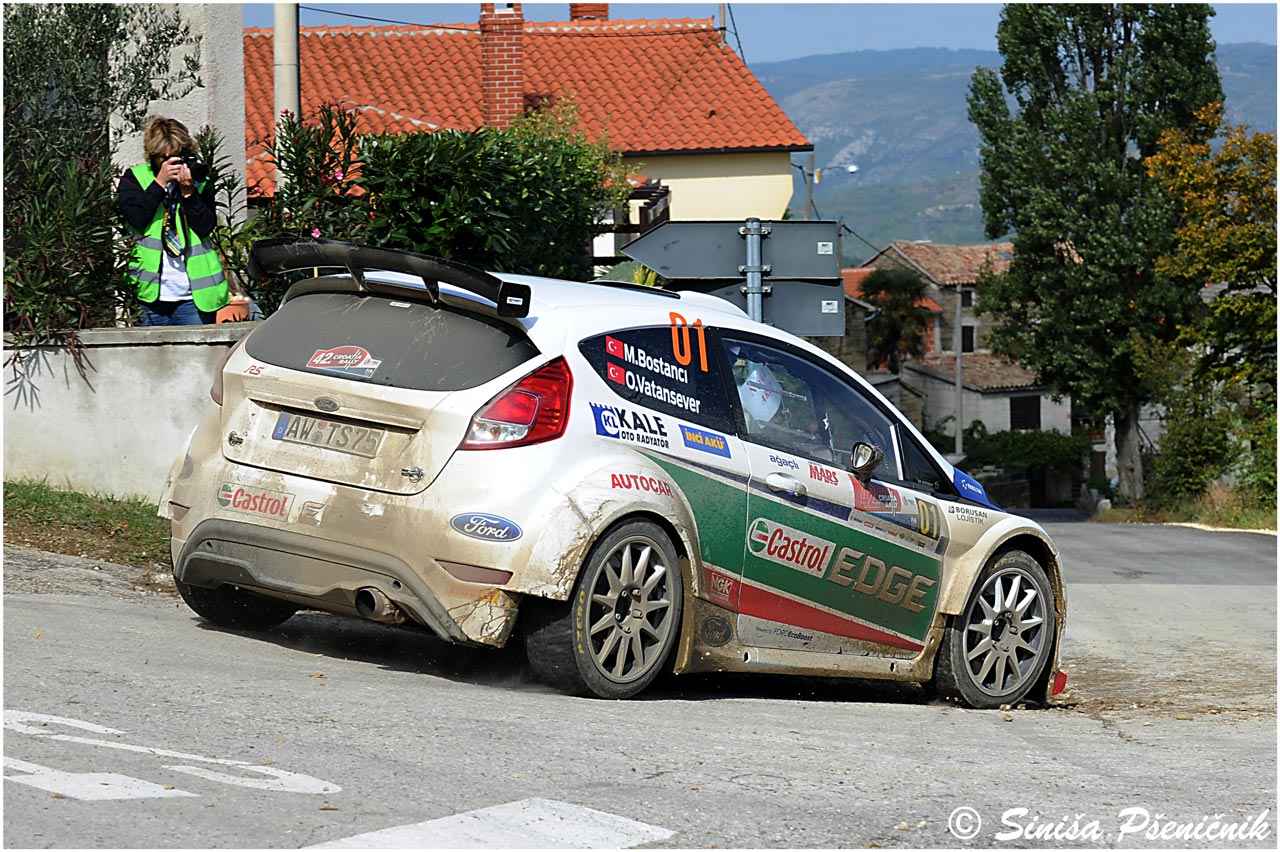This photograph captures a white Ford Focus rally car adorned with extensive branding and sponsor stickers, notably featuring large green and red Castrol Edge decals on its side. The car, labeled with the number 01 in orange, also displays a Ford sticker on the rear right and additional branding like "Castrol" on the rear left. Two red Turkish flags with white moons and stars are visible on the top left side. The rear quarter panel window carries the names of the drivers, M.BOSTANCI and O.VATANSEVER. The car is equipped with a wide body kit, large wheels, and low-profile tires. The scene is set in a residential neighborhood with big trees and a house with a clay-tiled roof. Mountains loom in the background. A person in green visibility gear, standing off to the side, is capturing the scene with a camera. The car’s state of motion is ambiguous – it could be stationary or moving, which might depend on the shutter speed of the camera used. The European location is suggested by a license plate marked with a blue line and the number AWTS75.